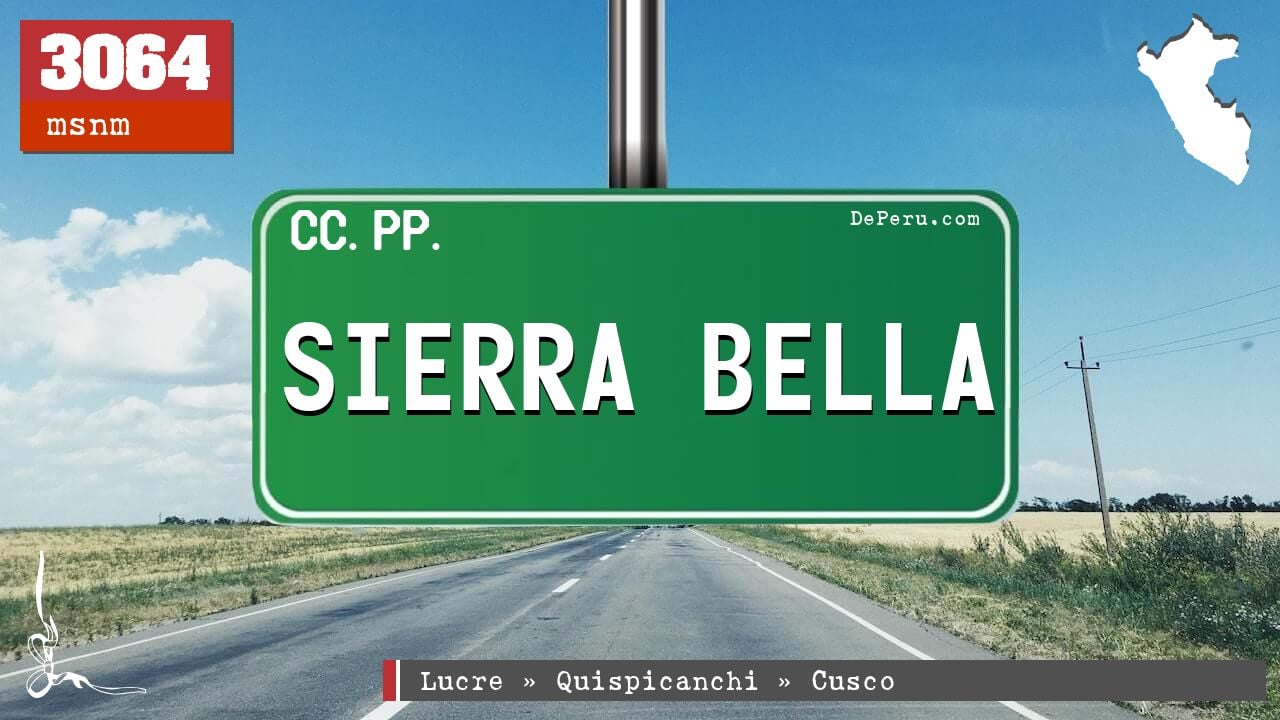The image captures a clear, bright day on a desolate two-lane highway flanked by flat open fields, their grass largely brown and sparse. Telephone poles line the roadside, adding an element of isolation. Dominating the center of the image is a green highway sign suspended on a pole. The sign prominently displays "Sierra Bella" with additional inscriptions: "CC.PP." on the top left, and "DePeru.com" on the top right. At the bottom right corner of the image, text reads "Lucre, Kispikanchi, Cusco" in white letters on a dark gray background with a white and red trim on the left side. A red square with "3064 MSNM" in white is placed at the top left corner, while a portion of a map outline is visible in white at the top right corner. The sky above is a vibrant blue, dotted with white, puffy clouds, amplifying the sense of openness and solitude in this rural setting.